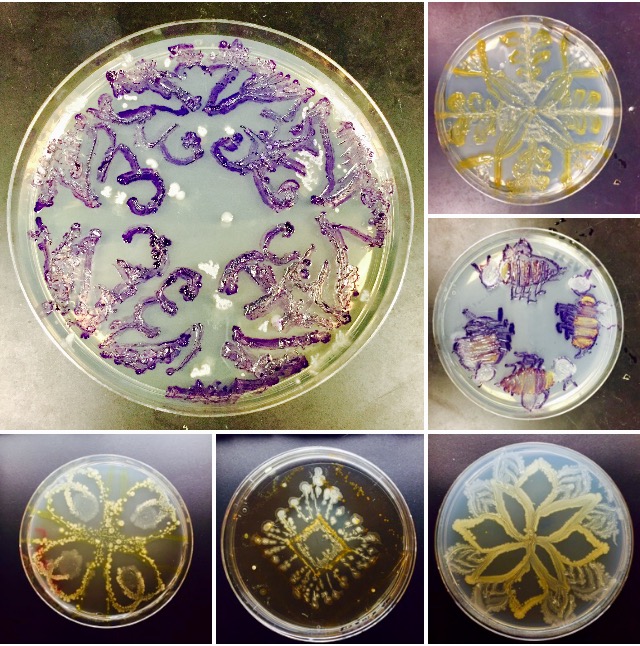The image showcases a collection of six distinct circular designs, arranged with one large central image in the top left corner and five smaller images aligned around it on the right side and bottom. The main plate at the top left features intricate purple patterns set against a cream-colored edge, strikingly similar to the effect of glitter set in glue. Each design, positioned within a white circle, contrasts against various backgrounds, predominantly shades of gray and tan. The first smaller image mirrors the large design but employs a gold hue. The following design incorporates a golden triangle set on a dark background. Another features a purple and yellow pattern that stands out prominently. One image displays a golden floral design on a dark gray, smoky background, while another, appearing to depict honeybees with white and blue stripes, is set on a white circle against a gray background. The final image in the sequence shows a translucent circle with an elaborate gold design, set against a purple background. The overall composition evokes the aesthetic of petri dishes with vivid, glitter-like growths, suggesting a biological or laboratory theme.